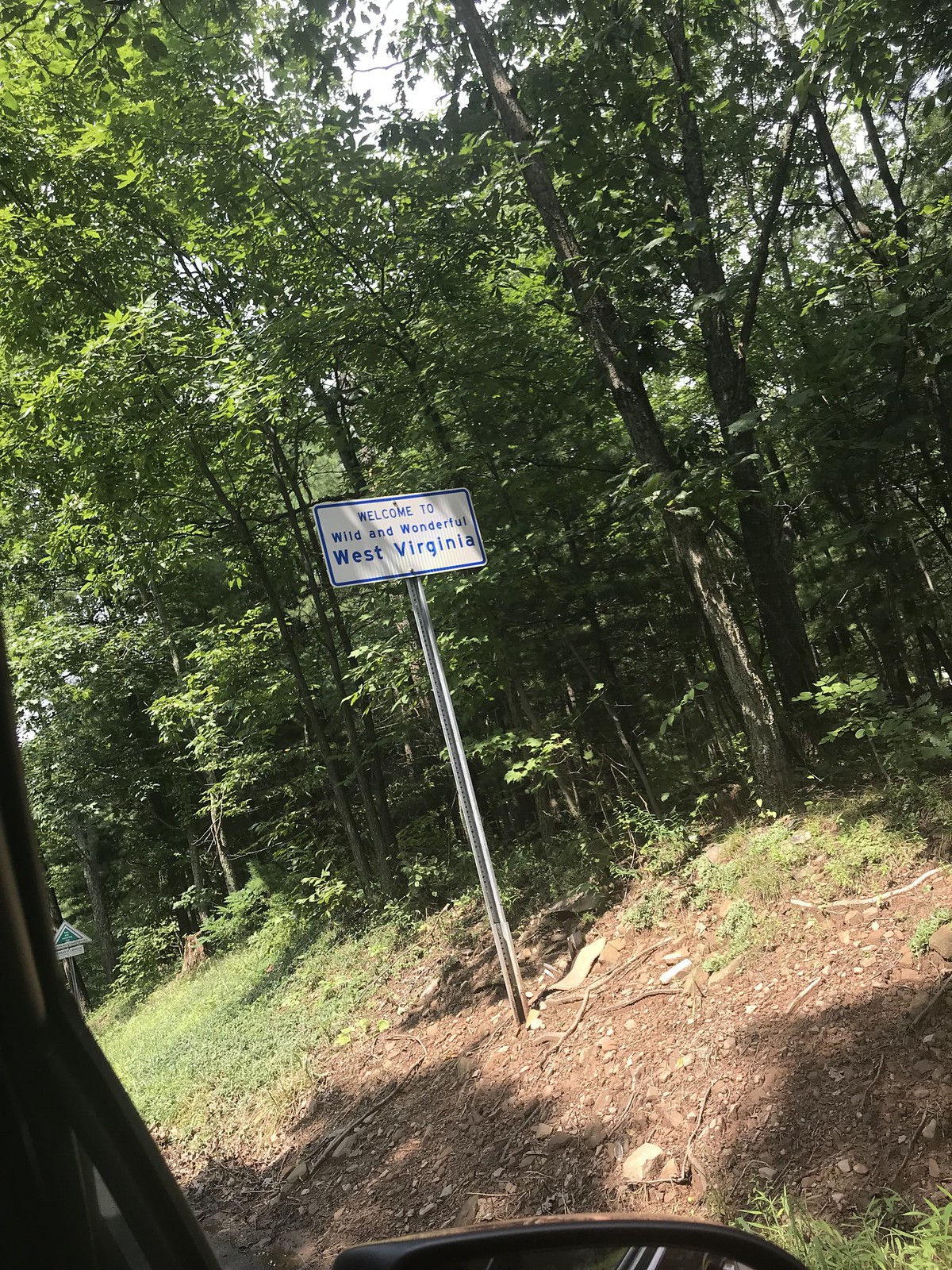The image captures the interior of a vehicle, which is likely a car or van, with a window view showcasing a serene outdoor landscape. Through the window, one can see an expanse of dirt and grass, leading to a dense area of tall trees that stretch upwards into a clear, light blue sky. The sunlight illuminates the scene, adding a warm, inviting glow.

In the far distance, there is a sign that is too distant to decipher clearly. Closer to the foreground, another sign is visible in the form of a white rectangle with its longer side aligned horizontally. This sign, written in medium dark blue text, reads, "Welcome to Wild and Wonderful West Virginia." The overall ambiance suggests a bright, sunny day, highlighting the natural beauty of the surroundings.